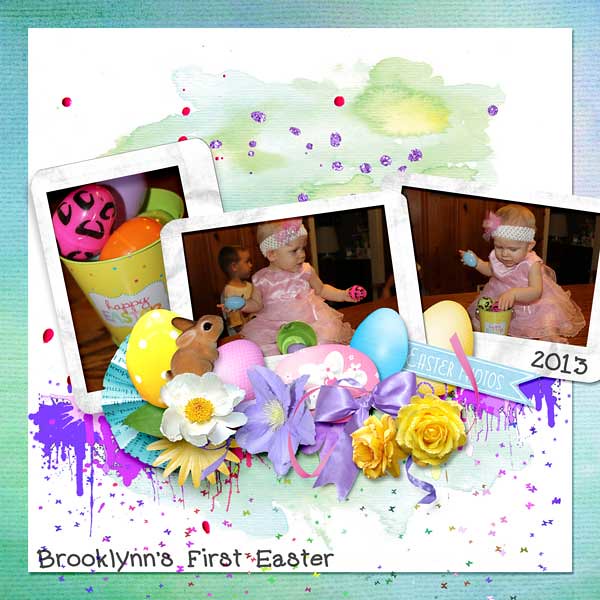The card celebrates Brooklyn's first Easter with three Polaroid-style photos, each featuring an Easter theme on a blue background. In the left photo, there’s a yellow cup filled with colorful Easter eggs. The middle photo shows a young girl, assumed to be Brooklyn, who is about one year old. She has no hair and is dressed in a satiny pink dress with ruffled trim and wears a white headband adorned with a flower. Brooklyn holds Easter eggs in both hands while standing in what seems to be a living room. The right photo captures Brooklyn placing eggs into the yellow cup. Surrounding the photos, the card is embellished with Easter elements such as flowers, eggs, and a brown bunny. The text "Brooklyn's First Easter" is displayed on the bottom left corner, while "2013" is marked on the bottom right. The background behind the photos includes watercolor-like splashes of purple and pink, adding to the festive atmosphere.